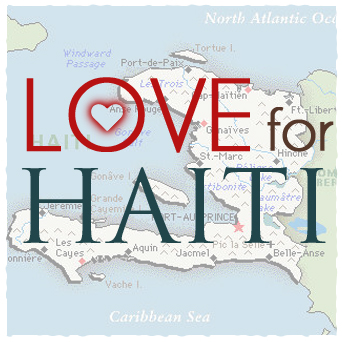The image is a small square photograph showcasing a map of Haiti, which is slightly faded but still legible, depicting the country's location in the Caribbean Sea and the North Atlantic Ocean. The map features various cities, including Les Cayes, Aquin, Jacmel, and Belle-Anse. Superimposed on this map is the phrase "Love for Haiti," with "Love" rendered in red lettering and a heart symbol within the 'O', while "for" is in brown text and "Haiti" is in dark blue text. The letters are large and dominate the center of the photograph, creating a strong visual emphasis on the message of love for Haiti amidst the geographical depiction of the island.